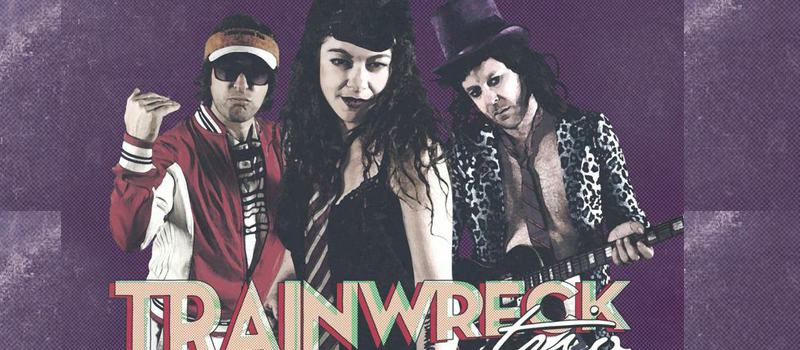Promotional art for the musical group Trainwreck features three prominently positioned individuals against a horizontally-oriented, purple background with various shades of dark and light purple smudges suggesting a dynamic backdrop. Across the bottom of the image, the band's name "TRAINWRECK" is displayed in large, all-caps letters with an orange-yellow color, outlined with red shading. Although partially cut off, cursive white text below potentially reads "trio," indicating the type of group.

The man on the left dons a red and white tracksuit-style jacket, hard-edged sunglasses, and a brown-and-white hat, with his right hand posed defiantly. He gives off a vibe of a middle-aged punk enthusiast, adding a bold flair to his appearance. The central figure, a woman, is closer to the viewer and sports long, wavy black hair. She is dressed in a sleeveless black tank top with lace detailing, a black necktie, and dark lipstick, exuding a mysterious and edgy presence. Something black on her forehead may be a mask or hat, though it is indistinct. To her right stands another man, distinctive in his flamboyant attire of a purple top hat and a leopard print jacket left open to reveal his bare, hairy chest. He holds a guitar and has a black necktie hanging loosely around his neck, further emphasizing the band's eccentric and bold style.

This vivid and detailed scene captures the essence and persona of Trainwreck, offering a glimpse into their dynamic and eclectic visual identity.